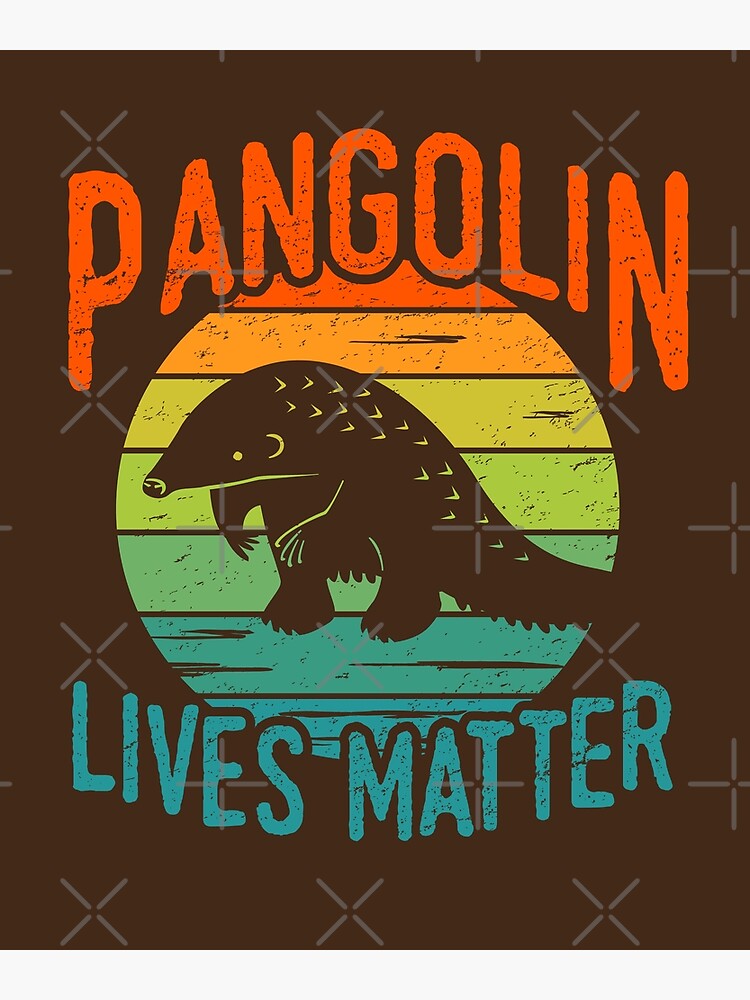The image appears to be a graphic design likely intended for a poster or t-shirt. It prominently features the phrase "Pangolin Lives Matter," a possible reference or parody of the Black Lives Matter movement, emphasizing the importance of pangolins. The text "Pangolin" is rendered in orange, while "Lives Matter" is in blue or turquoise, both in a retro or distressed style to give a worn look. At the center, there is a detailed drawing or silhouette of a pangolin in brown, positioned in front of a circular gradient background that transitions from red and yellow at the top to green and blue at the bottom, resembling a sunset. The entire design has a brown backdrop adorned with light gray X's, plus symbols, and small white stars, possibly watermarks to prevent unauthorized use. The overall image is rectangular and taller than it is wide, with what looks like a wooden floor in multicolored hues of orange, yellow, and blue beneath the pangolin. This detailed composition makes up the engaging visual presented.